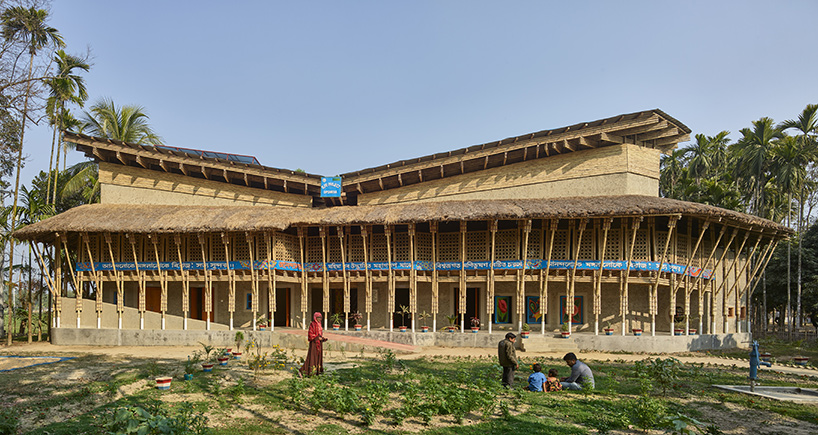The photograph captures a serene, sunny day in front of a striking two-story building designed to resemble an older Tibetan temple, despite its modern construction. The exterior of the building features a combination of tans and browns, with gentle V-shaped, inward-curving roof peaks and small flying buttresses supporting a grass-covered roof. The open-air structure reveals some artwork through its exposed sections. Palm trees frame the scene on both sides, under a clear, medium-blue sky. A woven blue banner is threaded through the middle of the building, adding to its unique aesthetic.

In the lush green foreground, which includes a mix of grass and weeds, a picturesque family scene unfolds. A woman dressed in a red sari with a red headscarf is walking toward the right, where a family appears to be having a picnic on the grass. The family consists of a seated man, a standing woman, and two small children who are also sitting on the ground, all facing away from the camera. To the right, a concrete pad holds a blue hand pump, hinting at the blend of old and new in this setting. The overall atmosphere is peaceful and semi-modern, enriched by the backdrop of palm trees and clear sky.